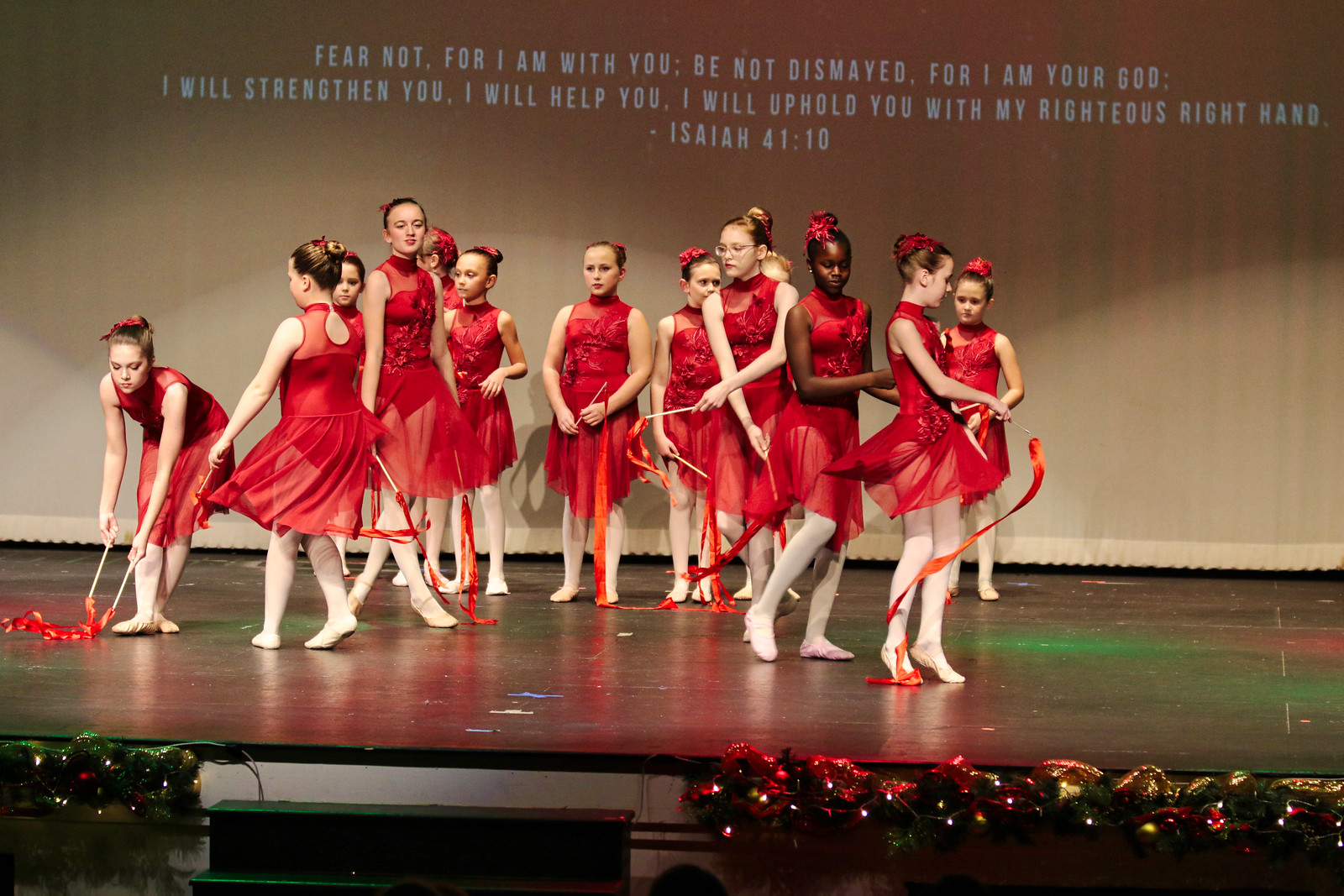In this evocative real-life photo of a ballerina dance recital, a group of approximately 10 to 15 young girls are captured mid-performance on a wooden stage. Their outfits uniformly consist of elegant red dresses reaching their knees, complemented by white leggings and ballet shoes. Adorning their hair are matching red ribbons, adding a delicate touch to their ensemble. 

The girls are equipped with sticks attached to flowing fabrics, reminiscent of ribbons or streamers, which they wield gracefully in various stances. One girl on the left is bent over, sweeping her streamers on the ground, while another girl beside her faces backward, directing her movements toward the first. Several other girls hold their streamers at their sides, with hands resting low.

The scene is beautifully set against a brown curtain, which bears an inspiring and reassuring biblical quote from Isaiah 41:10 in shining white letters: "Fear not, for I am with you; be not dismayed, for I am your God. I will strengthen you, I will help you, I will uphold you with my righteous right hand." The message is split across three lines and is prominently displayed, framing the performance with a sense of divine encouragement.

Adding to the festive atmosphere, Christmas lights in hues of red, green, and gold are strung across the front of the stage, twinkling warmly and complementing the performers' attire. The steps leading up to the stage are visible at the bottom of the image, grounding this enchanting scene in a poignant moment of youthful artistry and faith.